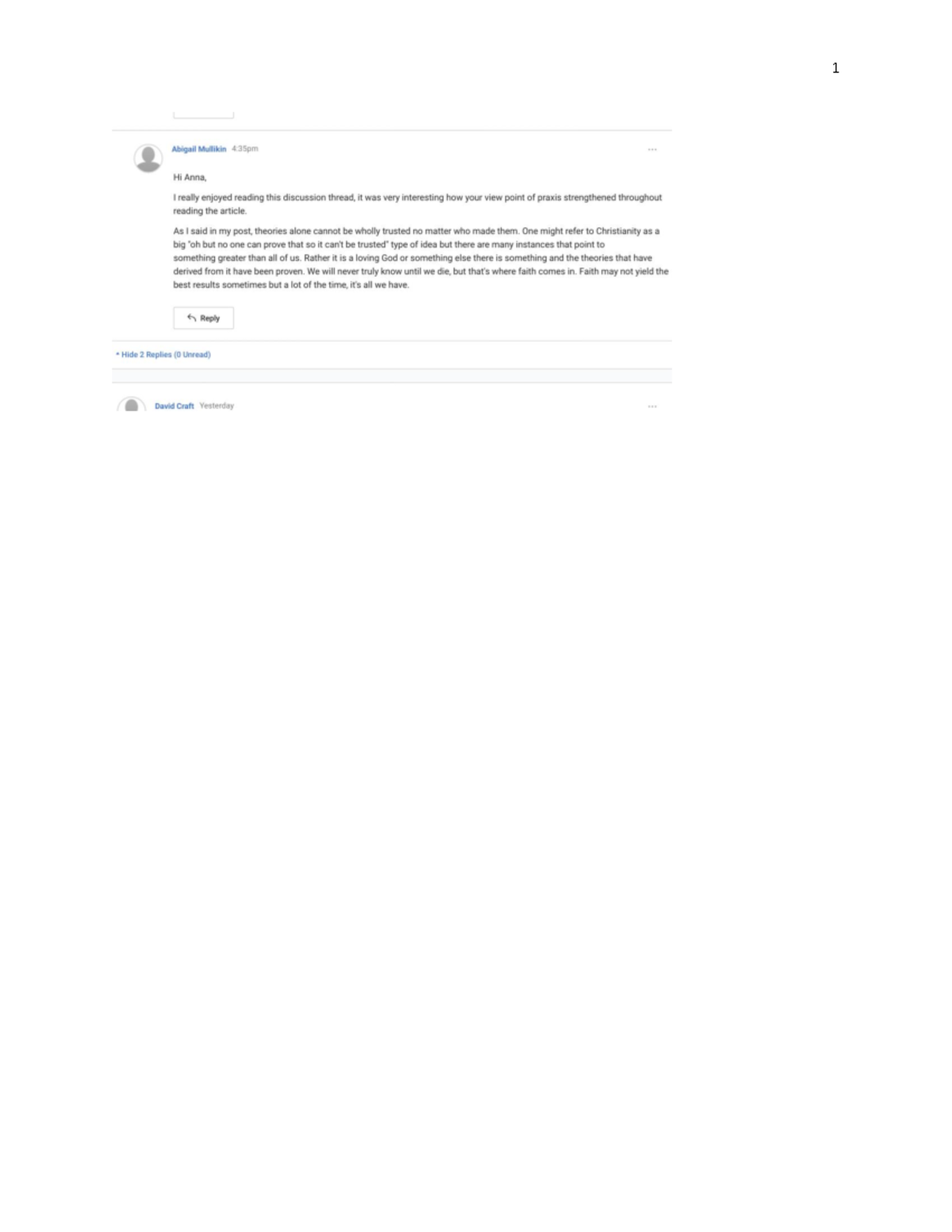The image displays an email interface with a predominantly white background. At the top, there is a horizontal grey line stretching from left to right. Below this line, a grey silhouette of a person is visible. Adjacent to the silhouette, in blue text, is the name "Abigail McCulkin," followed by an unreadable grey timestamp. The email appears to be from "Annabelle McCulkin," as indicated by the sender's details. The body of the email begins with a greeting, "Hi Anna," and continues with a message expressing how the sender enjoyed reading a discussion thread and found various viewpoints interesting. The email discusses the skepticism towards theories, regardless of the source, mentioning Christianity and the concept of faith. The text further highlights the sender's perspective on faith not always yielding the best results but often being the only thing people have. The remaining text is mostly unreadable but conveys a critical tone regarding religious beliefs.